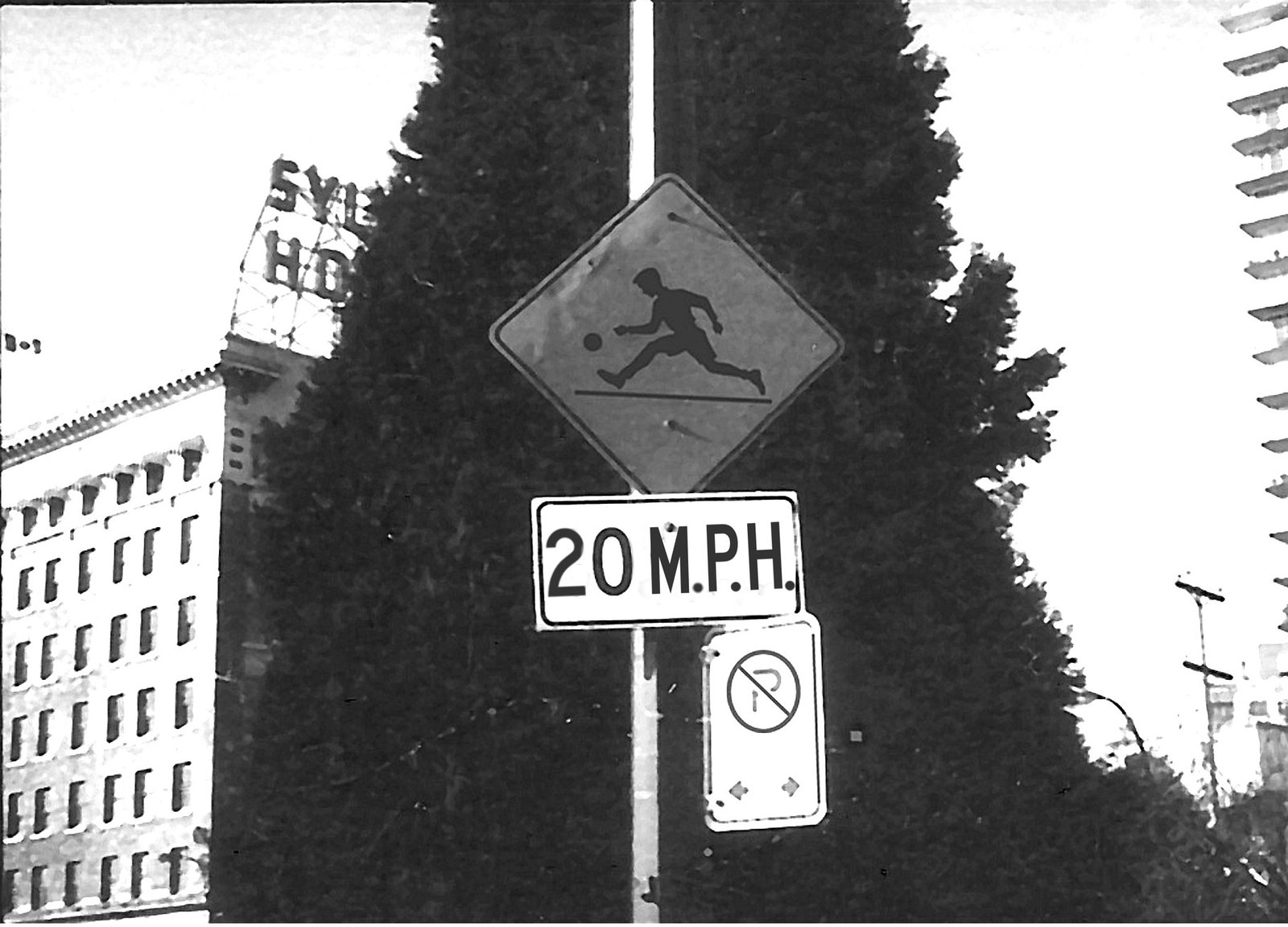In this black and white photograph, dated perhaps from the 1950s or 1960s judging by the architectural style and general ambiance, the scene presents a nostalgic urban landscape. On the left side of the image, a tall brick or block building towers over the street. While the faded scaffolding obscures part of the sign at its top, enough letters are visible to read "SYL" with the letters "HO" just below. This structure appears to be a hotel or a business of some kind.

On the right, an imposing apartment building stretches skyward, indicative of a high-rise development. Below, the middle ground of the photograph captures a secondary building and what seems to be utility poles, blending into the backdrop of city life.

Central to the image is a large, leafy tree standing majestically in the background. Prominently in the foreground, a white pole is mounted with a distinctive, rectangular sign. The sign features a silhouette of a boy running to the left as he kicks a ball. Positioned beneath, a white street sign bordered in black clearly reads "20 MPH," indicating a speed limit. Further down, a smaller white sign with a circled 'P' crossed by a slash, combined with two horizontal arrows, denotes a no-parking zone across this stretch of the street. Together, these elements encapsulate a moment frozen in time, offering viewers a glimpse into a bygone era of urban life.